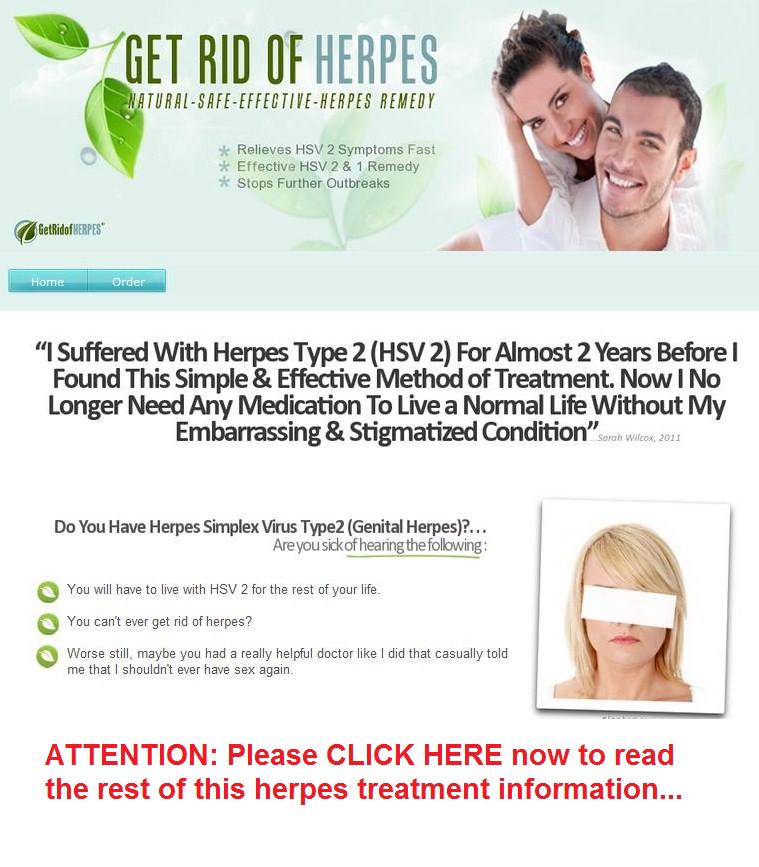The image is an advertisement from a website promoting a natural and safe remedy for herpes. At the top of the advertisement, two green leaves adorned with dew drops set a fresh, natural tone. The prominent headline reads, "Get Rid of Herpes: Natural, Safe, Effective Herpes Remedy."

Below this, a smiling couple is featured; the woman has brown hair, and the man, also with brown hair, has a light amount of facial hair. Both look directly at the camera, exuding confidence and happiness.

The central part of the advertisement highlights three key benefits of the remedy with star icons: 
1. "Relieves HSV2 Symptoms Fast"
2. "Effective HSV1 and HSV2 Remedy"
3. "Stops Further Outbreaks"

Further down, teal buttons for "Home" and "Order" are positioned on the left side. A heartfelt testimonial follows: "I suffered with Herpes Type 2 (HSV2) for almost two years before I found this simple and effective method of treatment. Now, I no longer need any medication to live a normal life without my embarrassing and stigmatized condition."

At the bottom, a woman's image is partially obscured by a white rectangle over her eyes, and a red print caption urges viewers, "Attention: Please click here now to read the rest of this herpes treatment information..."